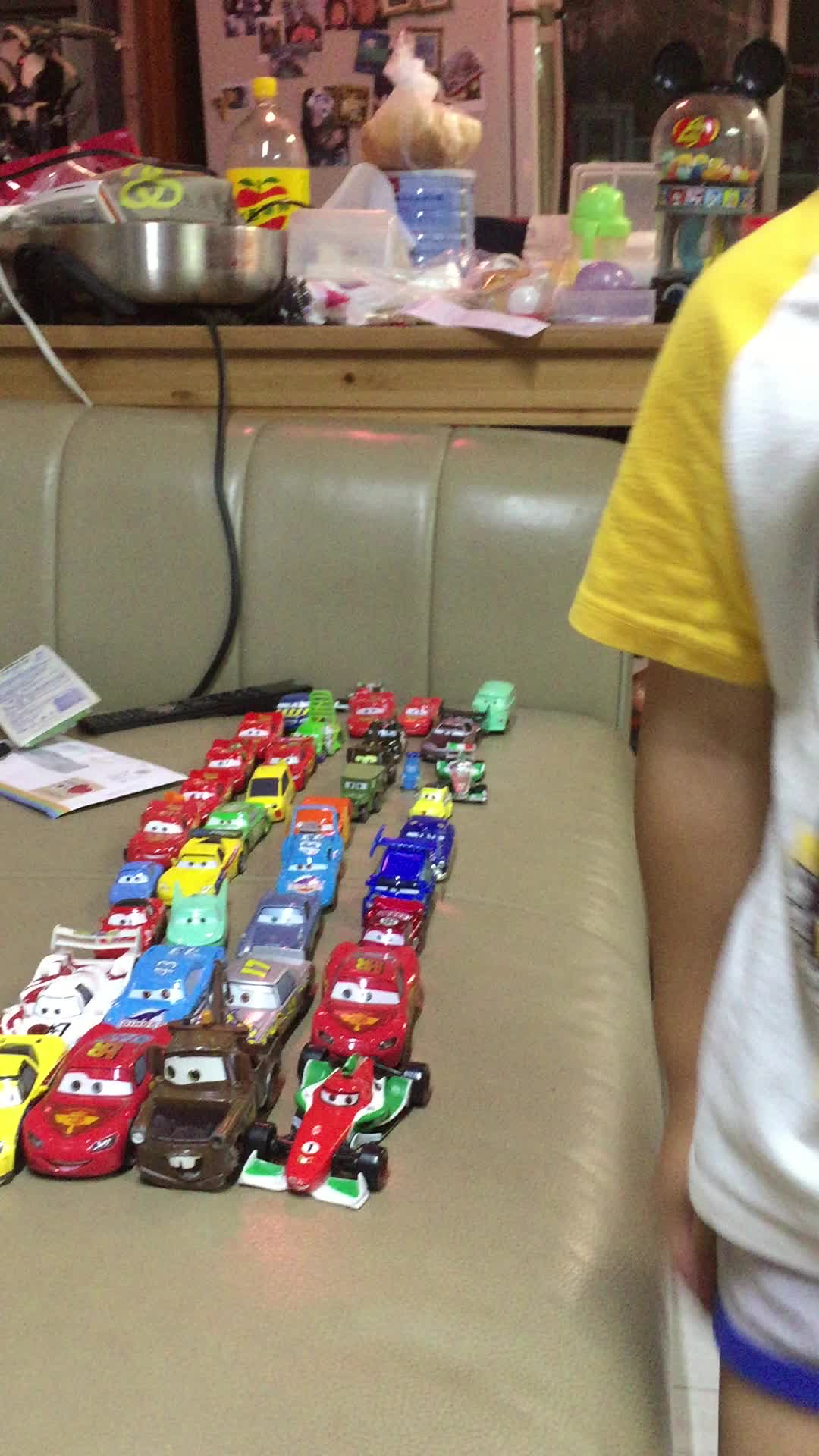The image depicts a collection of toy cars meticulously lined up in four vertical rows on a light gray, possibly tan-brown, couch. The toy cars, reminiscent of those from popular animated movies like "Cars," feature distinctive characteristics such as painted smiles and eyes on their windshields, indicating they belong to a common family despite their varied forms, which include trucks, jeeps, and racing cars. Notable cars include the brown tow truck and the red Lightning McQueen, with other cars showcasing a range of colors including red, yellow, blue, green, and black. On the left corner of the couch, two white pieces of paper and a hanging cord are visible, leading to a cluttered light brown table filled with various objects. A partially visible person stands to the right in a white shirt with a yellow sleeve and white shorts with a blue stripe. The background reveals a somewhat disordered kitchen worktop with bottles, aluminum containers, Tupperware, and an assortment of other items, as well as a couple of paintings adorning the walls.